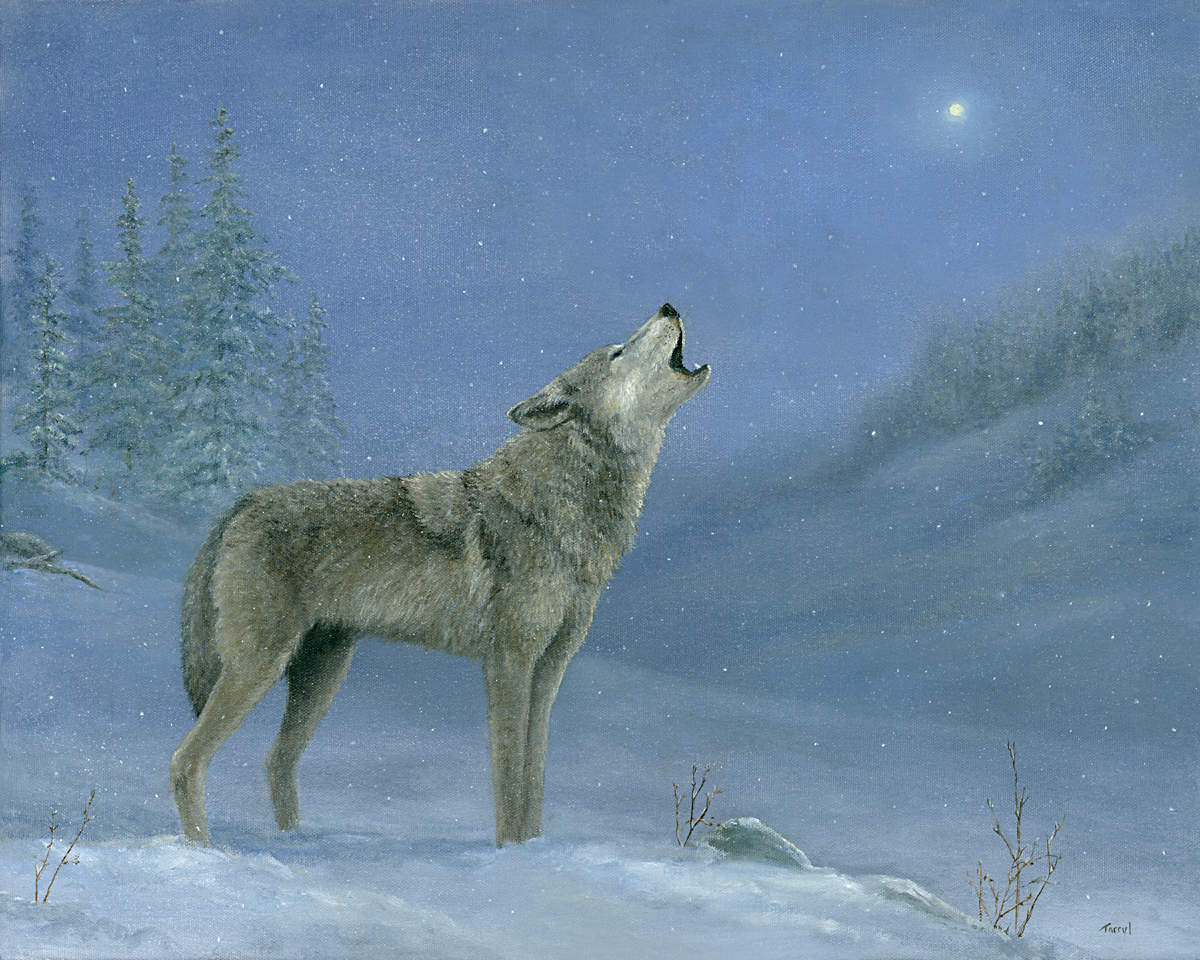The image depicts an intricate painting of a grayish-black wolf howling at a small, glowing moon, positioned in the upper right corner. The wolf, adorned in various shades of gray with a slightly lighter face, stands prominently on a vast, snow-covered landscape. Its head is tilted upwards with its mouth open in mid-howl, facing towards the right side of the painting. Below its feet, the icy ground stretches out, leading to a small stone in front of the wolf. In the far background, the left side features several tall, conifer trees coated in snow, standing sharply against the blurred, snowy trees on the opposite side. The snowy terrain further extends into a slope beneath the moon. You can also perceive faint textures of the canvas, emphasizing the painting's detailed brushwork and composition.